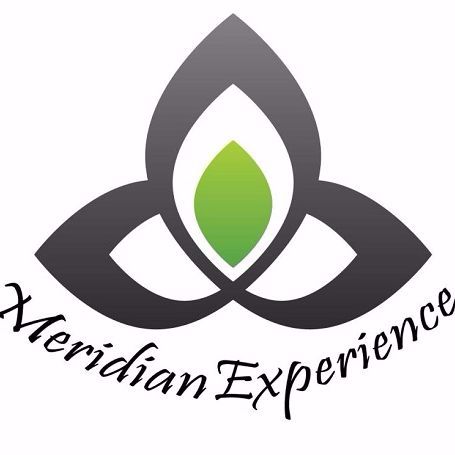The image depicts a detailed logo with a floral essence composed of three pointed oval petals arranged symmetrically: one petal points to the left, one to the right, and one straight up. Each petal has a thick gray outline and a white center, emphasizing the simple yet sophisticated design. At the heart of the upward-pointing petal, there is an additional smaller lime green pointed oval shape mimicking the larger petal's outline. Beneath the logo, the text "Meridian Experience" is displayed in a flowing cursive font, with the letters "M" and "E" elegantly capitalized. The overall background of the image is white, focusing the viewer's attention solely on the intricacies of the logo.